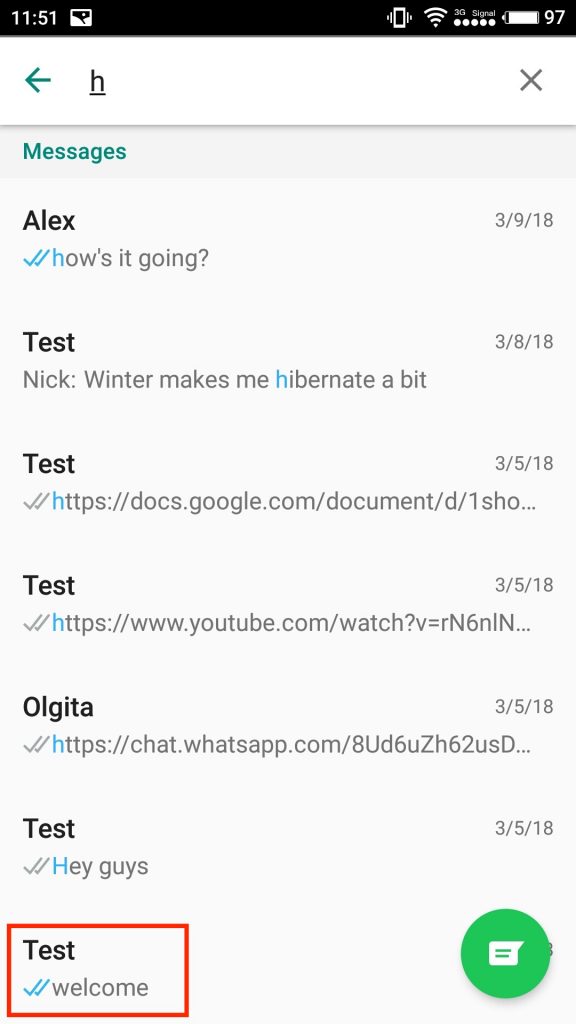This screenshot from a smartphone displays the time as 11:51 and shows the battery at 97% charge. Below the status bar, there is a turquoise arrow pointing left and a turquoise X button, both overlaid with the word "Messages." The screen lists various text messages in chronological order. The messages appear as follows: 
- "Alex: How's it going?" dated 3/9/18
- "Nick: Winter makes me hibernate a bit" dated 3/8/18
- A link to a Google Document, dated 3/5/18, labeled "test"
- A link to a YouTube video (https://www.youtube.com/watch?v=RN6NLN3) also dated 3/5/18, labeled "test"
At the bottom of the message list, the name "OLGITA" is displayed.